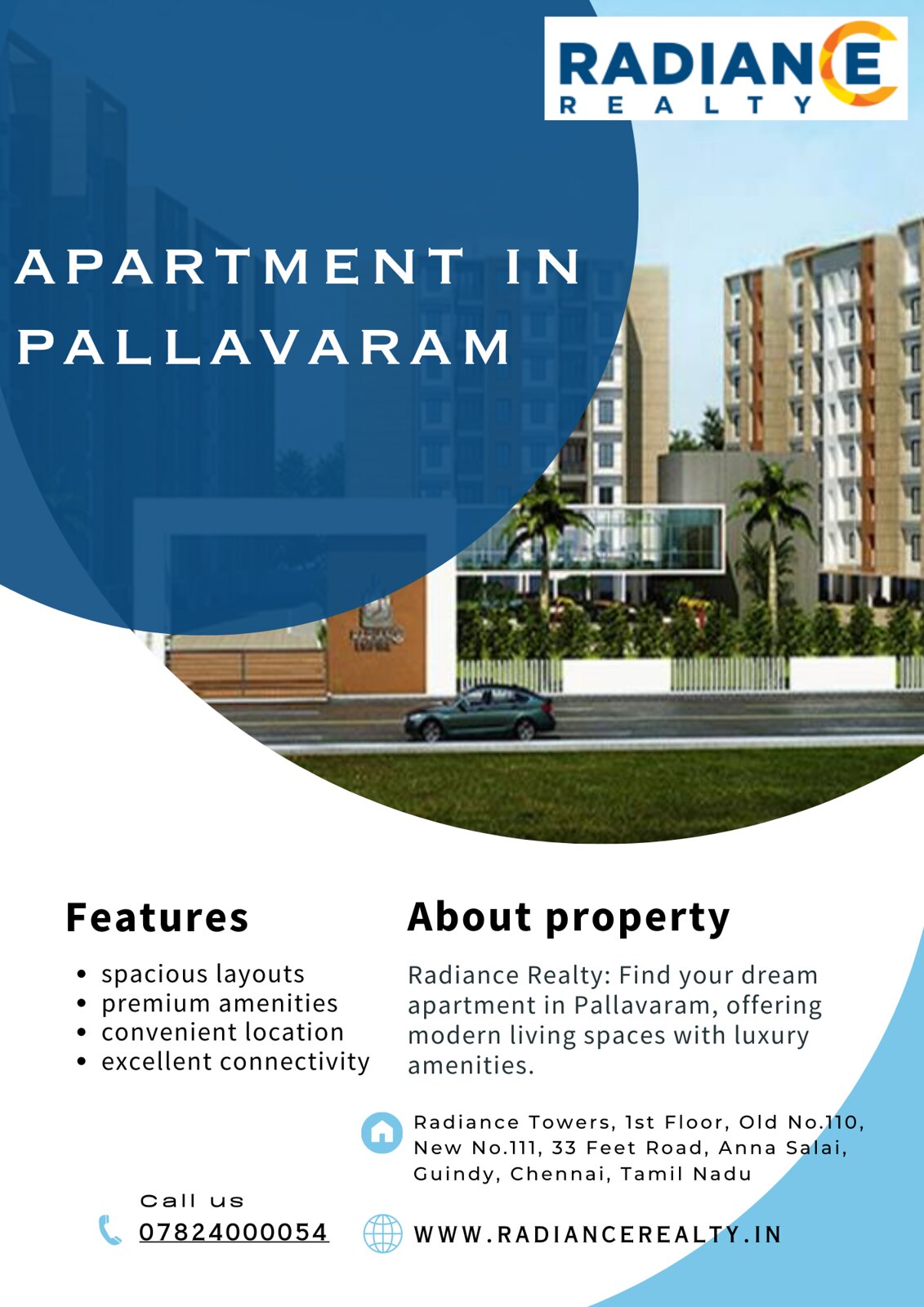The image is a detailed scan of a rectangular digital advertisement for Radiance Realty, which promotes an apartment in Pallavaram. The advertisement is taller than it is wide and features a mix of colors including blue, white, yellow, orange, green, brown, and black. In the upper right corner, "Radiance Realty" is prominently displayed with the letter 'C' enlarged and colored in yellow and orange, almost engulfing the letter 'E'. 

On the upper left side, there is a dark blue, slightly transparent circle containing the text "Apartment in Pallavaram." Below this, extending downward from the right upper corner, is another circle with an image depicting an apartment building, a car parked on the street in front, and tropical palm trees surrounding a small garden area.

The bottom half of the advertisement is primarily white, with a light blue section in the lower right corner. Important details about the property are listed in black print, under headings like "Features" which include bullet points: Spacious Layouts, Premium Amenities, Convenient Location, and Excellent Connectivity. Additional text provides further information such as, "About Property: Radiance Realty, Find Your Dream Apartment in Pallavaram, Offering Modern Living Spaces with Luxury Amenities."

Contact information is also provided: a phone number (078-2400-0054), a physical address (Radiance Towers, First Floor, Old Number 110, New Number 111, 33 Feet Road, Anna Salai, Gundee, Chennai, Tamil Nadu), and a website (www.radiancerealty.in). The overall design indicates a professional, modern living space ideal for prospective buyers looking for premium amenities and excellent connectivity.